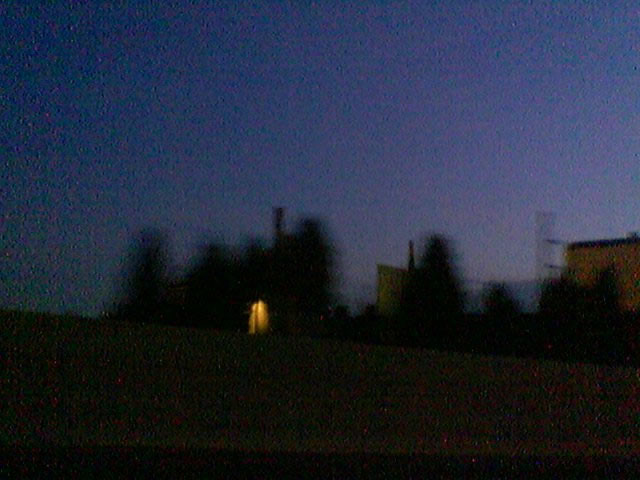A low-light, grainy image captures a twilight sky transitioning from deep blue at the top to a lighter hue near the horizon. A shadowy ground scene lies beneath the sky, with minimal details visible due to the darkness. At the forefront, a faint outline of what appears to be a low gray concrete retaining wall is discernible, though its identification is uncertain. Behind this wall, the silhouettes of dark-colored smokestacks or tall structures emerge, partially hidden by intervening trees. On the far right, a distinct yellow building adds a splash of discernible color to the scene. Centrally, just above the suspected retaining wall, a yellow light source, possibly from a porch or residential lighting, faintly illuminates the surrounding area, with little else visible beyond it.